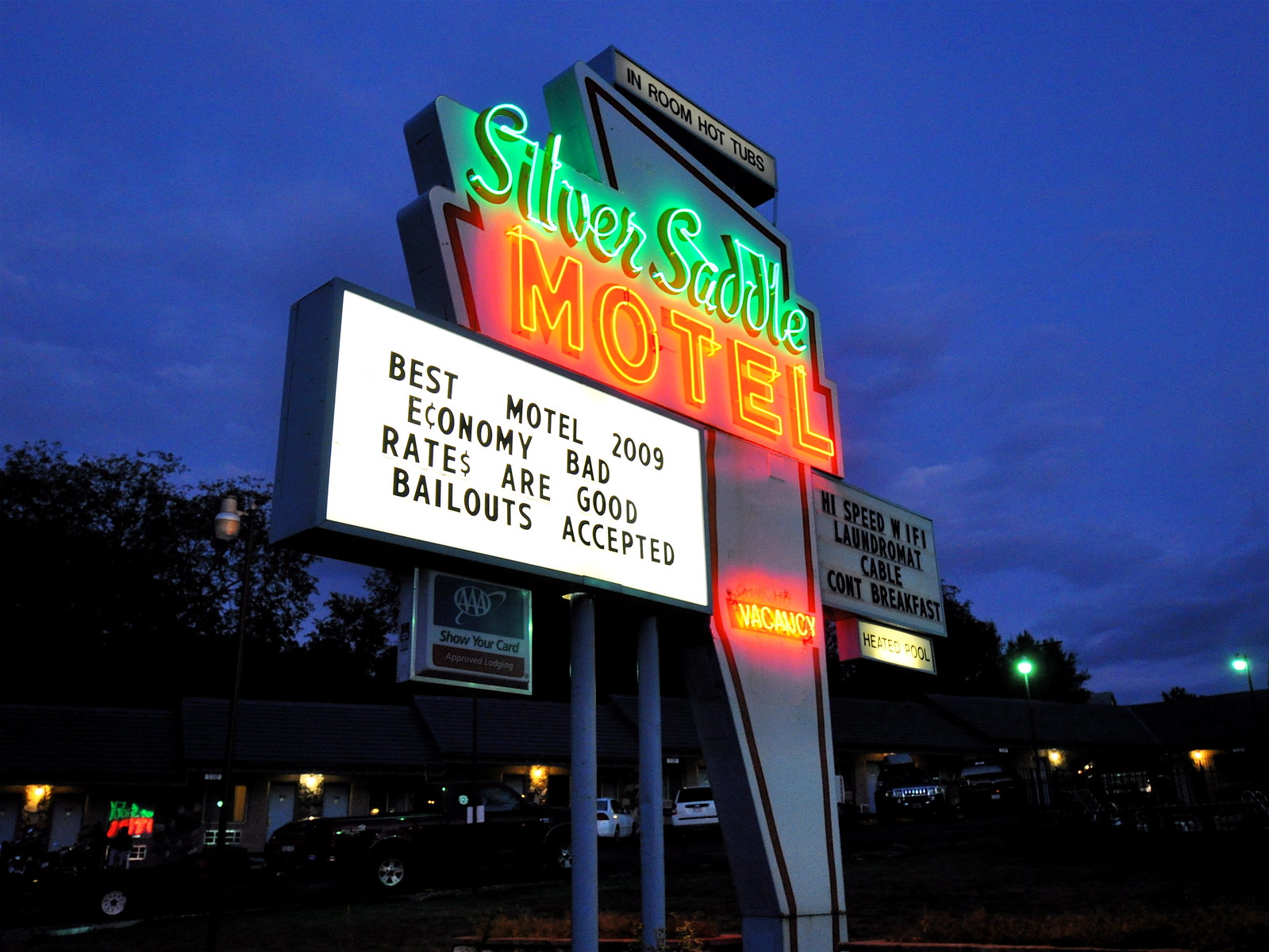In the image, there is a prominent sign in the middle depicting the Silver Saddle Motel, adorned with vibrant neon colors. The sign reads "Silver Saddle Motel" with "Best Motel 2009" displayed beneath it, followed by enticing offers such as in-room hot tubs, high-speed Wi-Fi, a laundromat, cable TV, and a complimentary breakfast. The words “Rates are Good” and “Bailouts Accepted” also catch the eye, along with a red "Vacancy" sign and an offer for AAA members to show their card for benefits. 

The scene is set outdoors, likely in the late evening or nighttime, with a clear dark sky above. Below the sign are rows of motel rooms with lights on, indicating occupancy, along with cars parked in front of the rooms. Trees border the top of the image, adding a touch of natural scenery to the background. The ground appears to be asphalt, suggesting a parking lot extending towards the bottom of the image. The overall atmosphere conveys a welcoming yet modest roadside inn with various amenities to attract travelers.